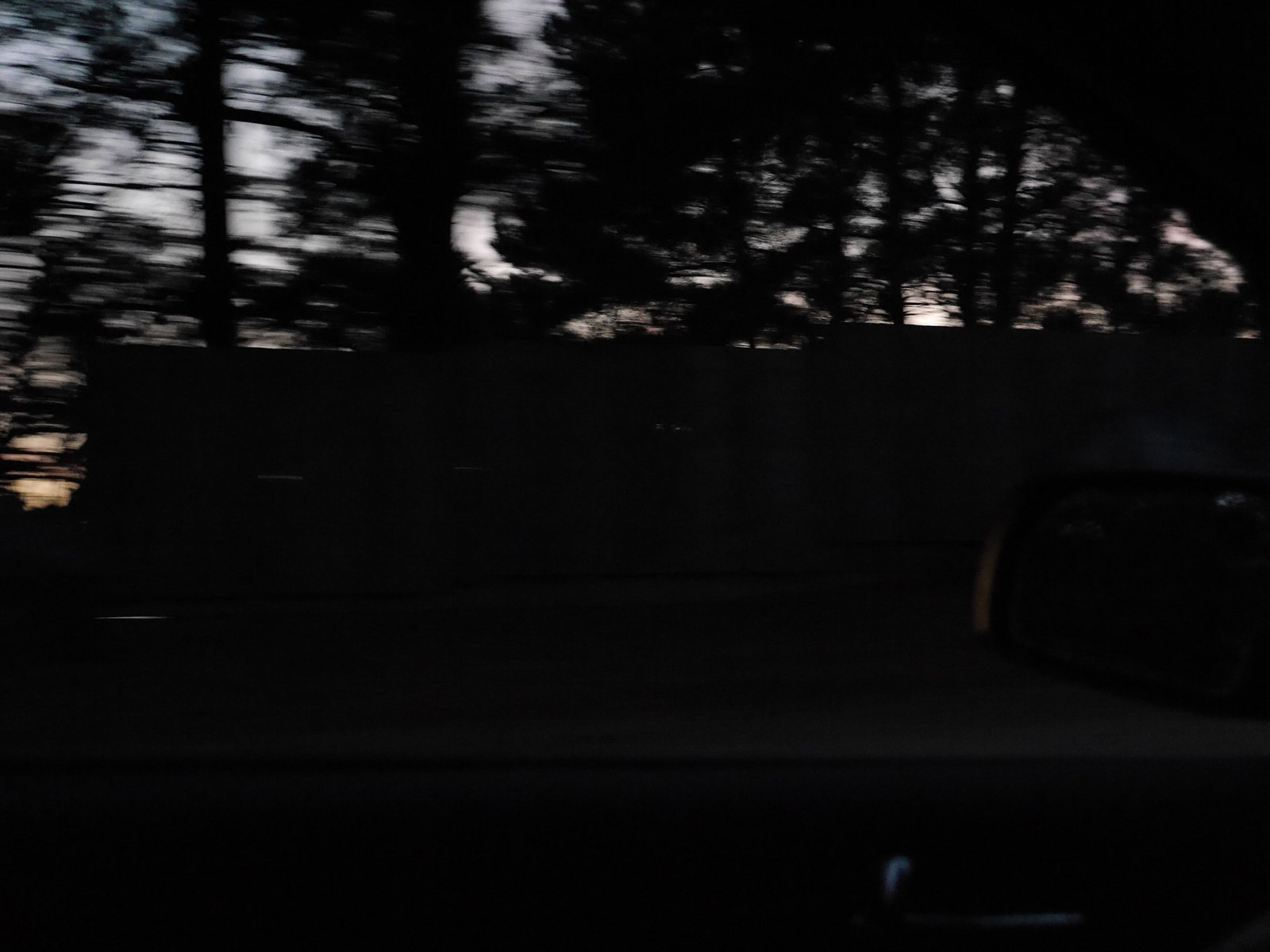The image appears to be taken outdoors at dusk, as the night is beginning to set in. The background features a gradient sky transitioning from light blue to light orange, suggesting a sunset. Silhouettes and outlines of numerous trees populate the scene, their leaves indicating it's spring or summer. These trees are especially dense on the right side, while the left side shows more detail with visible tree trunks and branches, allowing more light to seep through with a golden-brown hue. The bottom two-thirds of the image are mostly black, yet subtle streaks of color, including light blue and orange, appear near the right side. There’s a straight, horizontal line that might be the roof of a building, possibly viewed from a side mirror if taken from a car, contributing to the sense of motion and blurriness in the photograph. The environment depicted is dark and enigmatic, heavily shadowed with faint whispers of remaining daylight.